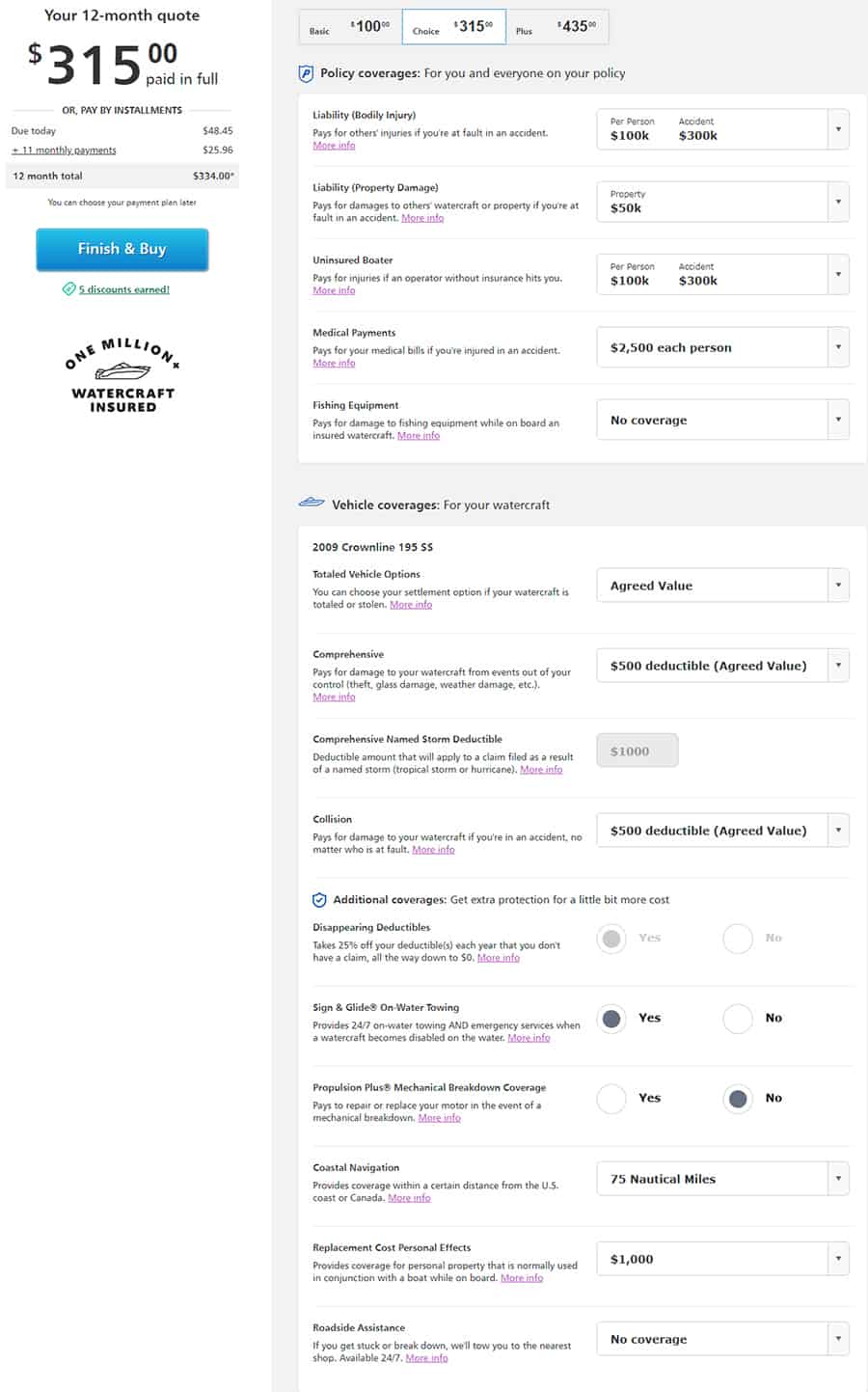Here is your cleaned-up and detailed caption:

---

The image depicts a comprehensive breakdown of a 12-month insurance quote for watercraft coverage. The total premium is $334, with an option to either pay $315 in full or opt for an installment plan with an initial due payment of $48.45 followed by eleven monthly payments of $25.96. Five discounts have been applied to the policy, which also notes that one million watercraft have been insured under this provider.

On the right side, policy options and coverages are detailed:

1. **Basic Coverage:** $100
2. **Choice Coverage:** $315
3. **Plus Coverage:** $435

The user has selected the "Choice" coverage option.

Under the "Choice" coverage, the policy offers:

- **Liability Bodily Injury:** Coverage amounts of $100,000 per person and $300,000 per accident, paying for injuries to others if the policyholder is at fault.
- **Liability Property Damage:** Coverage of $550,000 for damages to other watercraft or property if the policyholder is at fault.
- **Uninsured Boater:** Protection for injuries if hit by an uninsured operator, with $100,000 per person and $300,000 per accident.
- **Medical Payments:** Coverage for medical bills of $2,500 per person if the policyholder is injured in an accident.
- **Fishing Equipment:** Coverage for damage to fishing equipment while on board, although no specific amount is mentioned.
- **Insured Watercraft:** No coverage is provided for the policyholder’s own watercraft.

A "Finish and Buy" blue button is displayed, allowing users to finalize their purchase, and additional information is available for further details on each coverage option.

---

This version provides a structured, detailed, and coherent overview of the insurance quote information depicted in the image.